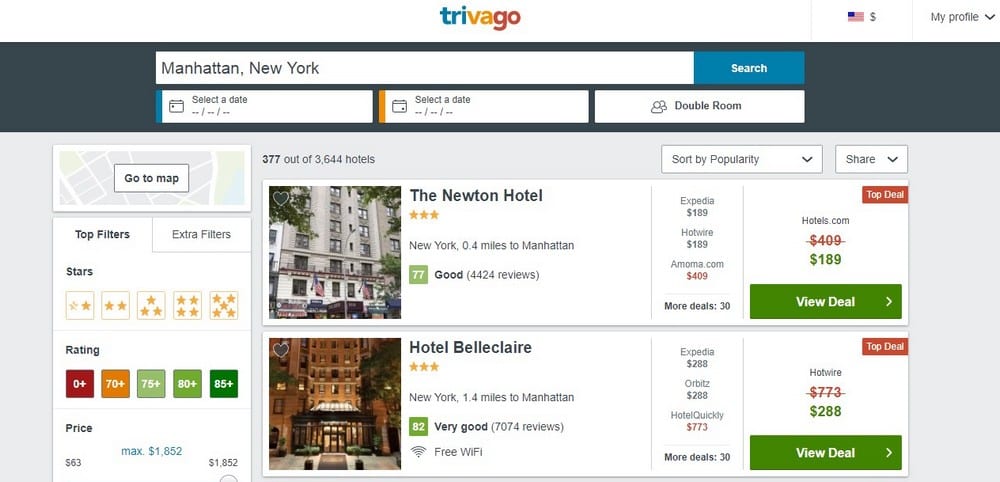The image is a screenshot of the Trivago website set to display in U.S. dollars. In the top right corner, there's a "My Profile" button. The search parameters are set for hotels in Manhattan, New York. No specific dates have been selected yet, and the search is for a double room. The search results show 377 out of 3,644 available hotels. 

The visible results include:

1. **The Newton Hotel**:
   - Rating: 3 stars
   - Distance: 0.4 miles from the center of Manhattan
   - Price: $189 on Expedia and Hotwire, with other sites listing it at $409
   - Features a green "View Deal" button
   
2. **Hotel Belcler**:
   - Rating: 3 stars
   - Distance: 1.4 miles from the center of Manhattan
   - Features: Free Wi-Fi
   - Includes a green "View Deal" button

Both hotels advertise significant discounts and have thousands of reviews, though the legitimacy of these deals is uncertain.